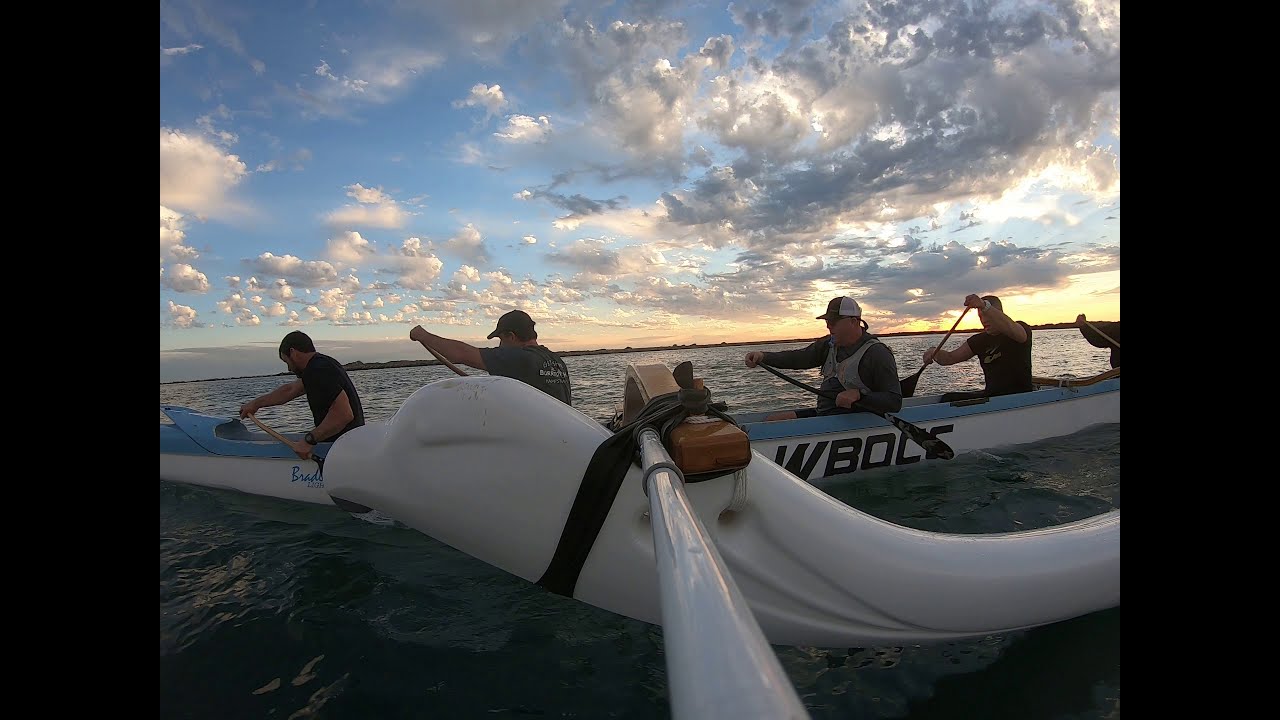The image depicts a group of five men rowing a boat on a calm ocean with a late evening sky overhead, partially filled with dark clouds. The boat, which appears to be a combination of two boats with a stick extending from the center, features a blue and white color scheme. The front part of the boat is blue while the bottom is white. There is a bit of cursive blue writing below the first rower, though it is hard to discern; however, "WBOC" followed by what might be another letter is visible below the third rower. The five rowers are seated in alternating positions: the first man on the left side with his oar, the second on the right, the third on the left, the fourth on the right, and the fifth visible man on the left, creating a synchronized rowing pattern to maintain the boat's balance. They are donning dark blue t-shirts, and the man in the center is wearing a life preserver vest.